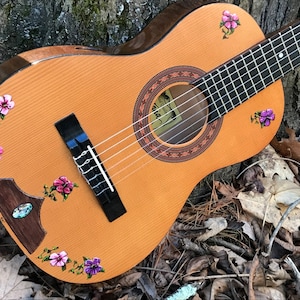This photograph captures the body of a wooden acoustic guitar, primarily occupying the frame, with the neck extending out of the upper right corner. The guitar's rich orange-brown wood showcases a fine, visible grain, and is adorned with dark purple and light purple floral appliques at both ends and small leaves intertwined with the flowers. Notably, a blue crystal gem is embedded towards the bottom center of the body. The guitar appears well-maintained and glossy, reflecting light, suggesting the image was taken on a sunny day. The background features a bed of dry leaves and sticks on the forest floor, with hints of vertical tree trunks and foliage. Bits of blue sky peek through in the upper left corner, adding to the natural outdoor setting.